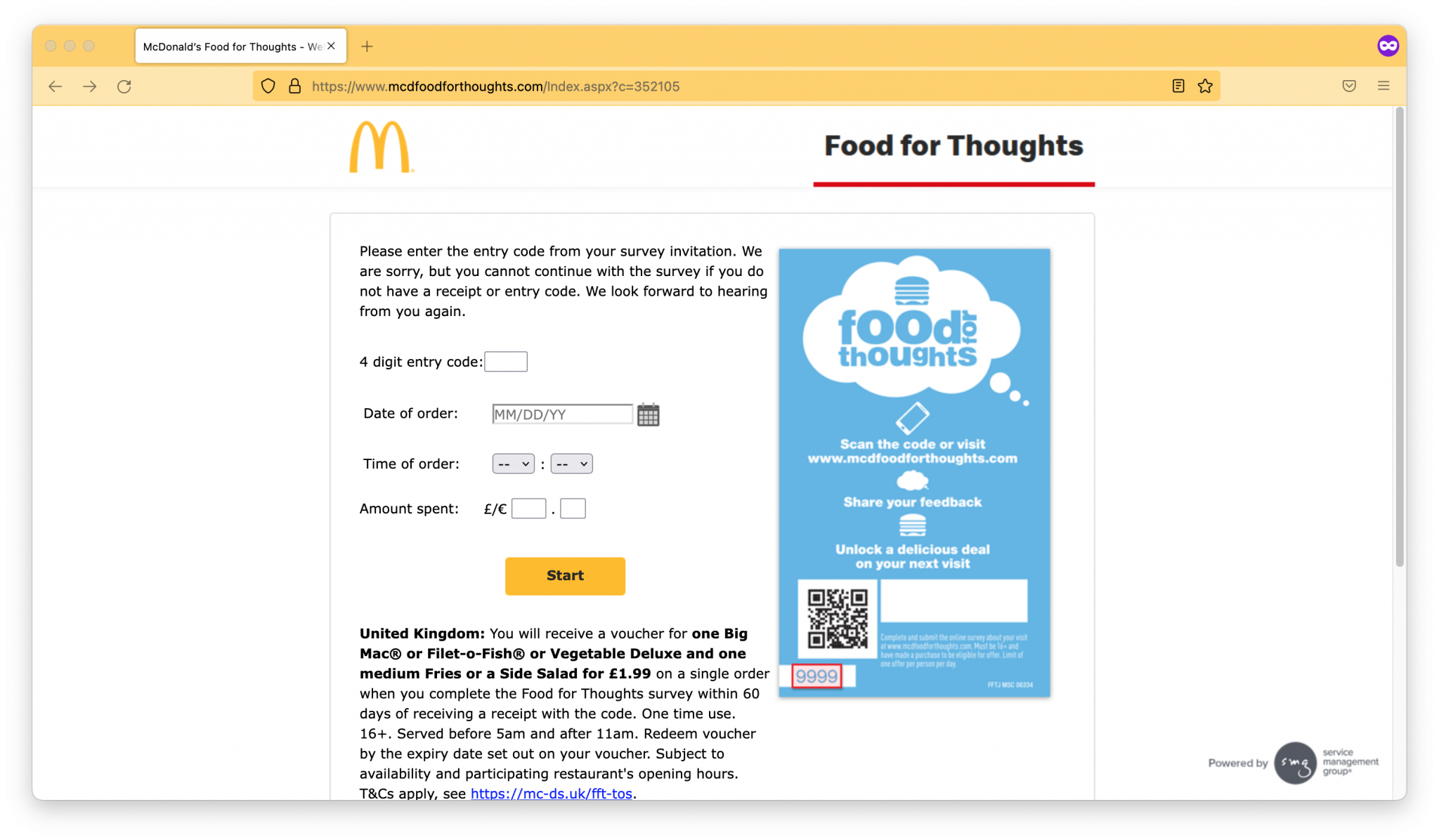The image showcases the McDonald's "Food for Thoughts" webpage, prominently displaying the iconic yellow 'M' logo at the top. The webpage URL is McDonaldsFoodForThoughts.com, with the phrase "Food for Thoughts" underlined in red beneath it. Below this header, the text instructs users to "Please enter the entry code from your survey invitation. We are sorry, but you cannot continue with the survey if you do not have a receipt or entry code. We look forward to hearing from you again."

The page features fields for a four-digit entry code, the date of order (with a calendar widget), the time of order, and the amount spent. There is a yellow "Start" button with black text for users to begin the survey process. At the bottom of the page, it states "United Kingdom," and details a promotional offer: "You will receive a voucher for one Big Mac or Filet-O-Fish or Vegetable Deluxe and one Medium Fry or a Side Salad for £1.99 on a single order when you complete the Food for Thoughts survey within 60 days of receiving your receipt with the code. One-time use, 16+, served before 5 a.m. and after 11 a.m. Redeem voucher by the expiry date set out on your voucher, subject to availability for participating restaurants' opening hours. Ts and Cs apply."

A link to the McDonald's webpage is provided in blue text. Additionally, the page features a "Food for Thoughts" icon depicting a hamburger inside a thought bubble, accompanied by blue text instructing users to "scan the code or visit www.mcdfoodforthoughts.com, share your feedback, unlock a delicious deal on your next visit." This section also includes a QR code and a red box displaying the numbers 9999, all set against a white background.